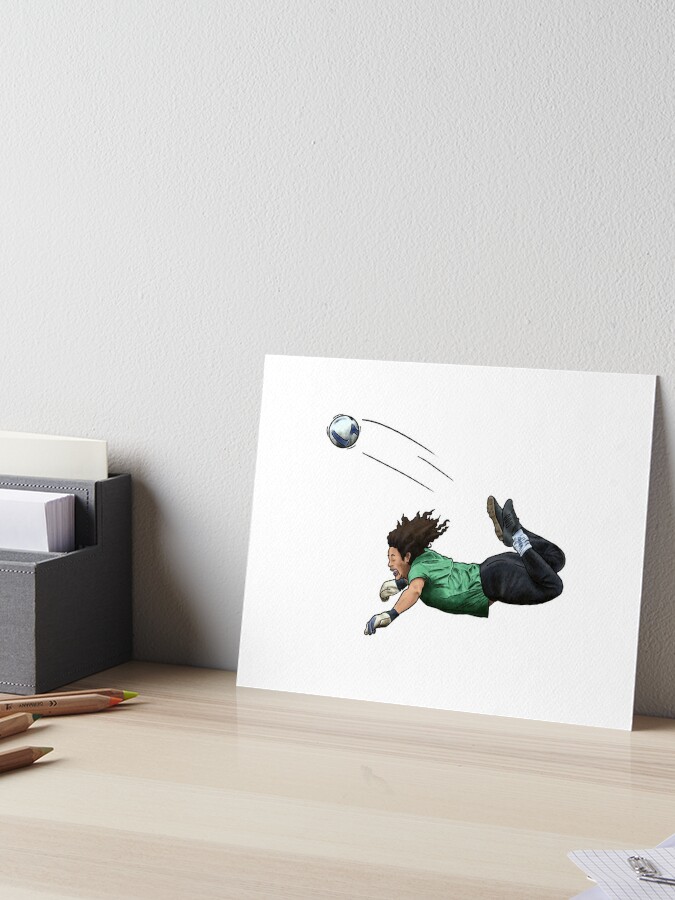The image displays a drawing situated on a light wooden table, positioned against a white, textured wall. The artwork, rendered on white construction paper, depicts a soccer player performing an acrobatic move, seemingly lunging forward and kicking a soccer ball mid-air with their back leg, indicated by motion lines around the ball. The player, with long, dreaded or curly brown hair and androgynous features, is attired in a green jersey, black pants, black spiky shoes, and white and blue gloves. The drawing is surrounded by wooden colored pencils, predominantly yellow and orange, and adjacent to it is a paper organizer containing more paper. This detailed scene suggests the drawing was recently completed, with art supplies still scattered on the table.